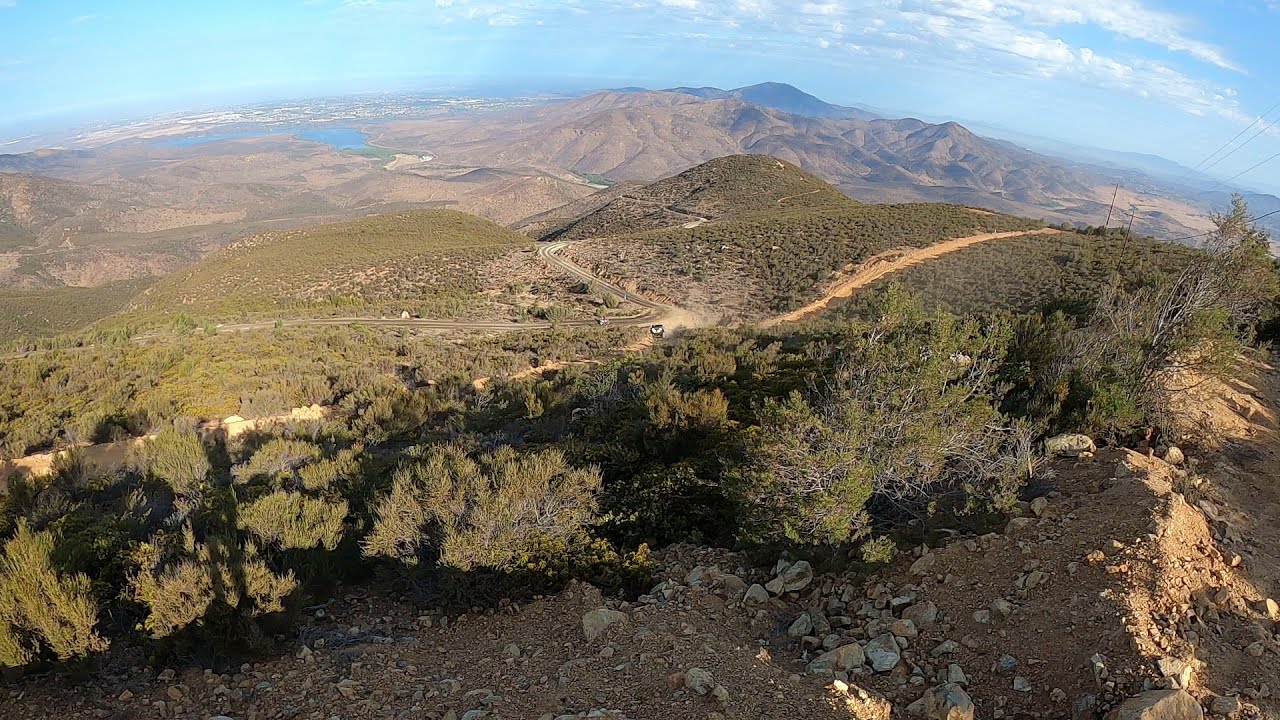This daytime outdoor scene captures a sweeping, hilly landscape dominated by rugged terrain and a series of undulating hills and mountains. The foreground prominently features broken stones and brown dirt interspersed with small, greenish shrubbery. Looking beyond this initial layer, several dirt trails wind through the scene, one of which has a car navigating its path. These winding trails and roads add to the dynamic feel of the landscape as they cut through the hills and lead towards the background.

In the mid-ground, thick brush and juniper bushes give way to a vast, hilly, and mountainous valley area. Roads meander through this undulating terrain, highlighting the region's rugged beauty. The hills and mountains in varying shades of brown and green stretch far into the distance, where a serene lake and possibly the outline of a city or town can be glimpsed. 

Above this intricate landscape, the sky spans a rounded strip at the top of the image. A tranquil blue sky, adorned with some white clouds, crowns the scene. On the right-hand side, the sky transitions to show a darker mountain edge below the clouds. Additionally, electrical lines can be seen hanging down on the right side, adding a subtle human element to the otherwise natural panorama. The entire composition exudes a sense of expansive, untouched wilderness.